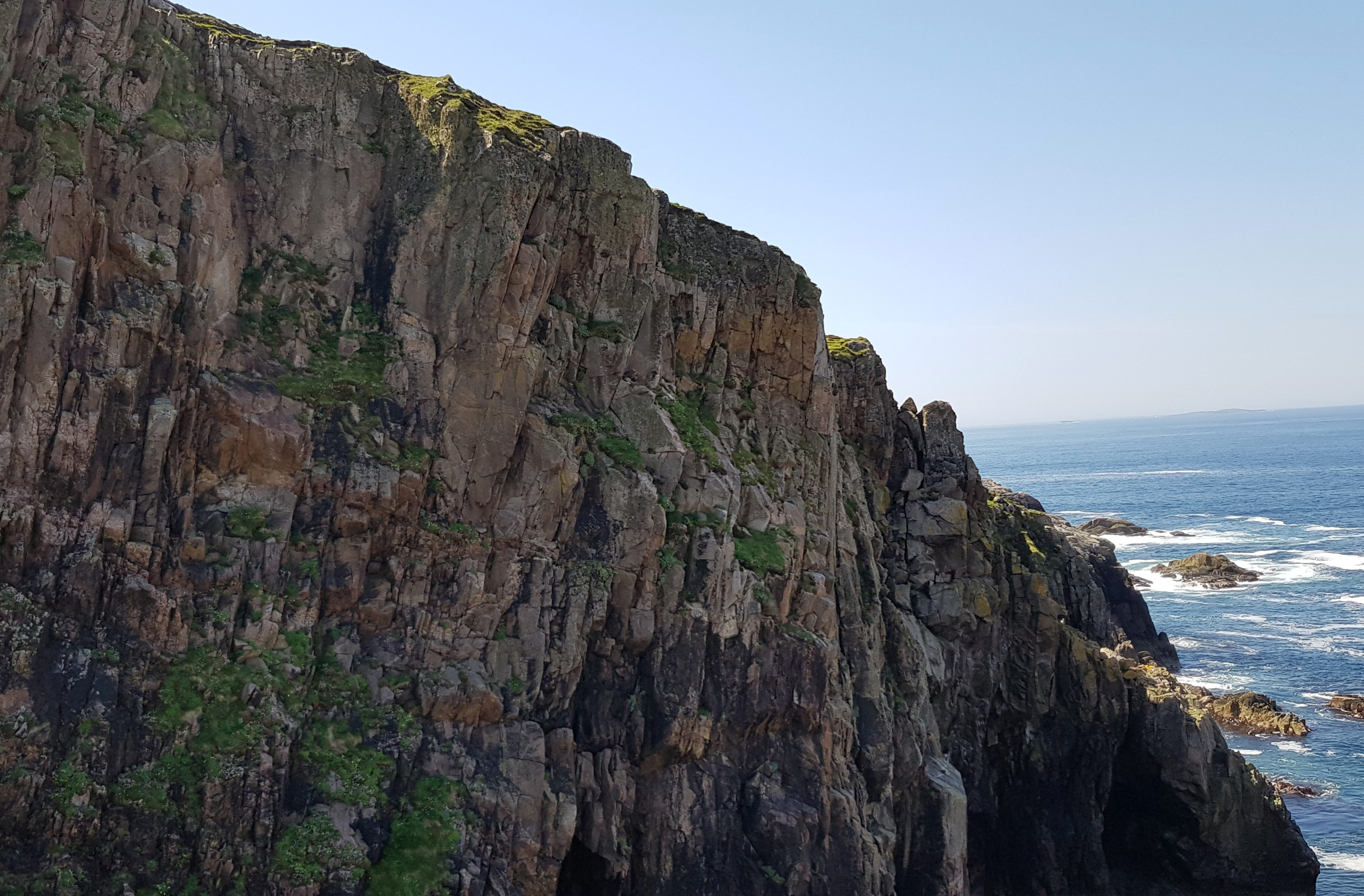The image depicts a rugged cliffside descending into an ocean. The cliff face, casting a shadow, features a myriad of colors including brown, orange, black, and gray, with patches of green vegetation sprouting from its crevices. The structure tapers gradually from the left side of the image down to the right, where it meets the expansive, blue waters of the ocean. In the sea below, several rock formations protrude from the water, surrounded by white ocean foam. The backdrop reveals a muted, bluish-gray sky with a hint of atmospheric perspective that gently blurs the distant vista. The presence of rocky land further in the background adds depth to the tranquil coastal scene.